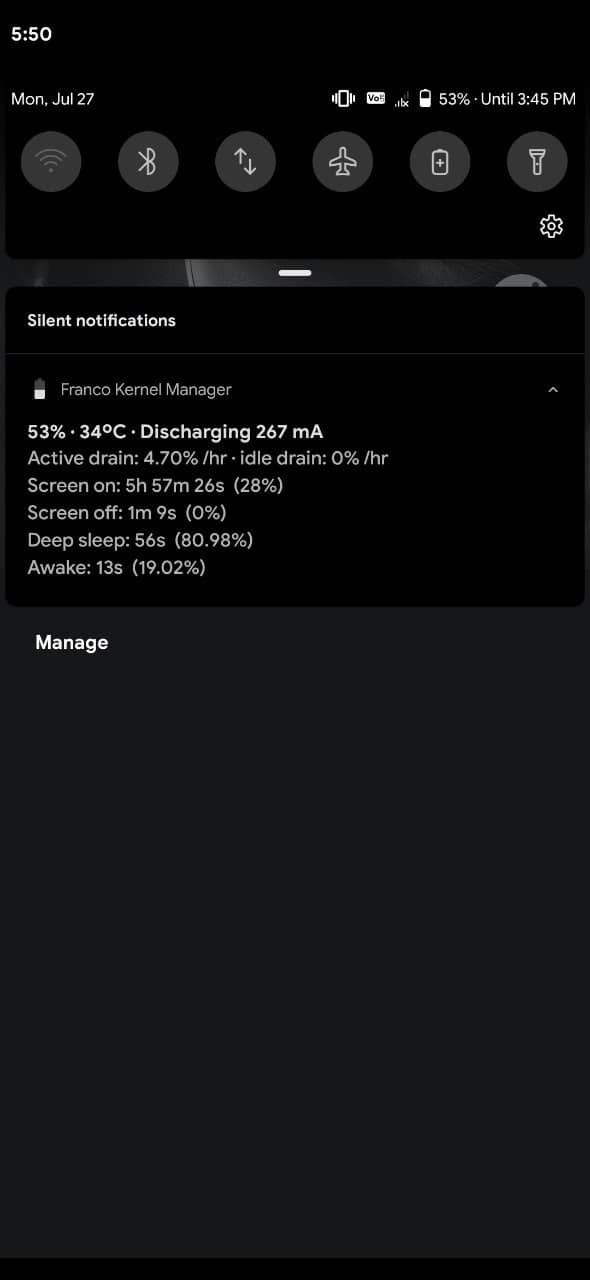The screenshot captured on Monday, July 27th, at 5:50 AM, shows a smartphone notification describing various device statuses and metrics. The phone is vibrating and displays a VOOS notification at 53% battery, estimated to last until 3:45 PM. WiFi is turned off, while Bluetooth is enabled. A grey circle with an airplane indicates that airplane mode might be activated. The image also shows icons for a battery, flashlight, and gear (settings). Silent notifications are active, and the Franco Kernel Manager app informs that the battery is at 53% with a temperature of 34°C, discharging at a rate of 267 milliamps, equating to an active drain of 4.70% per hour. The screen has been on for 5 hours, 57 minutes, and 26 seconds, consuming 20% of the battery, and has been off for 1 minute and 9 seconds. The phone has also experienced 56 seconds of deep sleep, accounting for 80.90% of the session, and 13 seconds of active use, tallying 19.02%. A grey notification labeled "Manage" is partially visible, with the user seemingly unsure about its specifics.